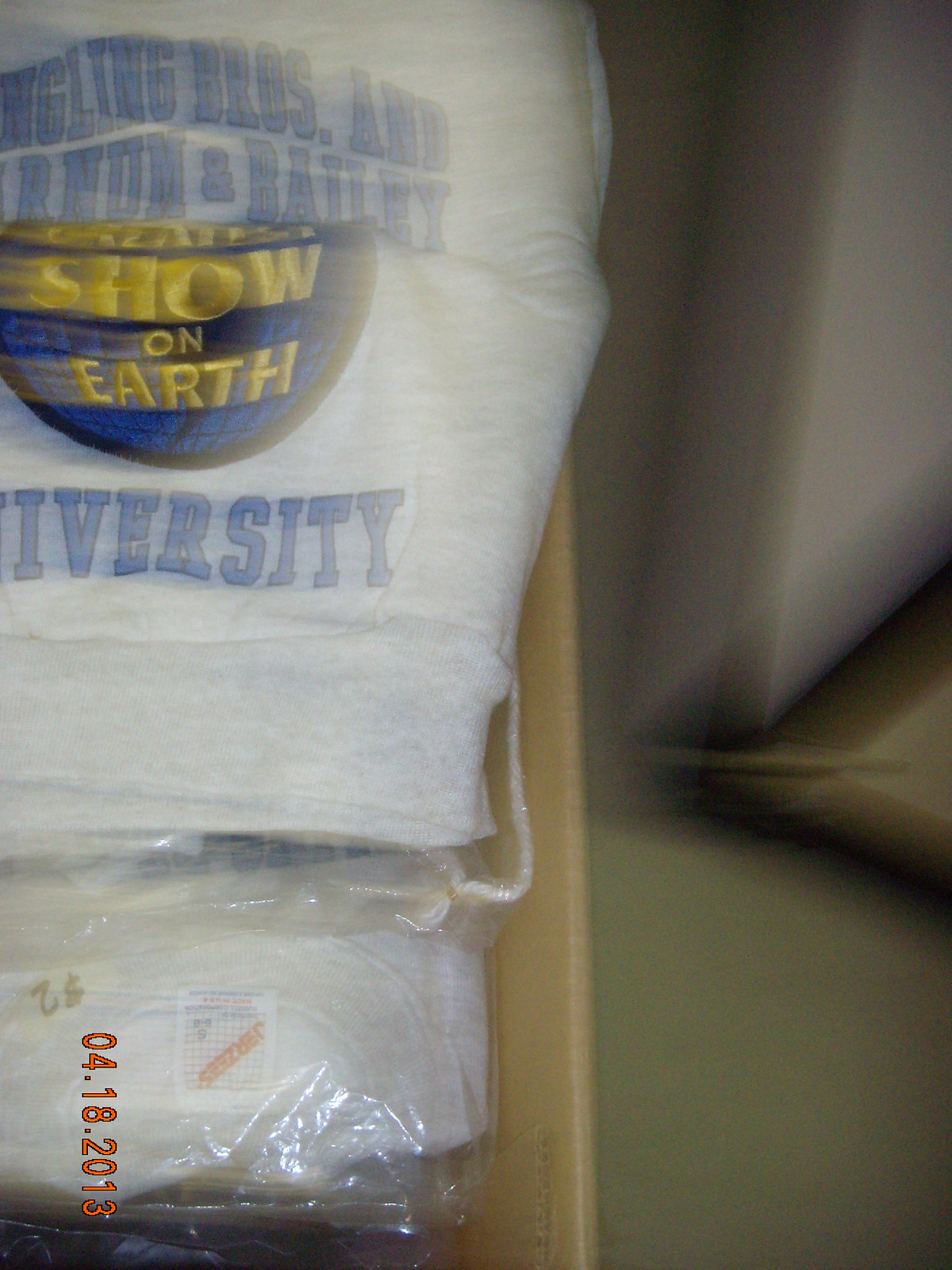This color photograph, taken indoors on 04-18-2013, is extremely blurry and turned sideways. The date stamp can be seen in red in the bottom left corner of the image. On the right side, a portion of a triangular-shaped object is visible. The left side of the image appears to show the inside of an open dresser drawer or a cardboard box, constructed from wood, containing various white cloth items.

In particular, there is a white shirt wrapped in plastic, with part of a tag showing. Above it, another white cloth item is prominently displayed, featuring blue text that reads "Ringling Bros. and Barnum and Bailey University," along with a globe logo that declares "Greatest Show on Earth" in gold. This logo is encased in a dark blue circle with a black border. Additional similar items wrapped in plastic can be seen, possibly towels or t-shirts, with some faint obscured text due to the blurriness.

Overall, the background remains unclear with what appears to be some additional indistinct boxes to the right, enhancing the sense of a cluttered storage area.